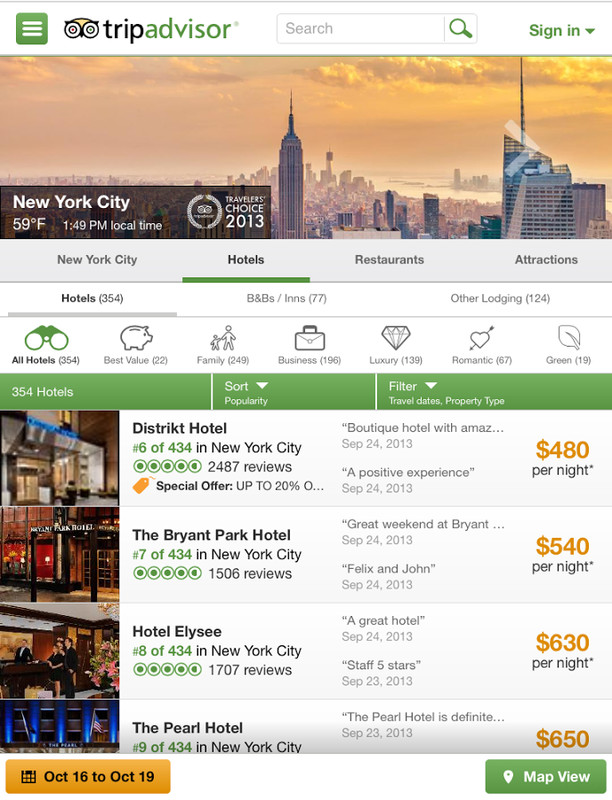This is a screenshot of a travel application showcasing various interface elements and features. At the top, the application sports a light gray header. On the left side of the header, there's a green square with rounded corners featuring a white hamburger menu icon. Adjacent to the hamburger menu is the application's logo, depicted as a cartoon owl's head with large eyes. The owl's head is yellow, with the left eye (from our perspective) containing a red dot and the right eye containing a green dot.

To the right of the logo is the title "TripAdvisor," where "Trip" is in black lowercase letters and "Advisor" is in green lowercase letters. Following the title is a white search bar with a thin light gray outline and slightly rounded corners. Inside the search bar, on the left side, is the placeholder text "Search" in light gray. On the right side of the search bar is a light gray square housing a green magnifying glass icon. To the further right, outside of the search bar, there is green text that reads "Sign In," accompanied by a dark green downward-pointing triangle.

Beneath the header is a thin green line that separates it from the main body of the page. The top portion of the body features a banner photograph, an aerial view of New York City with the Empire State Building prominently in the center against an orange cloudy sky. At the bottom left of this photograph is a translucent black rectangular pane with large white text that reads "New York City." Below this, in smaller white text, it displays "59°F" followed by "1:49 PM local time."

To the right of the temperature and local time information, there is a badge with the same owl logo, but in white. Surrounding the logo are two white laurels, and below it, it reads "TripAdvisor." Underneath the badge, in all caps on separate lines, it says "TRAVELERS' CHOICE 2013."

The remainder of the page shows hotel listings, although details of these listings are not described in the screenshot.